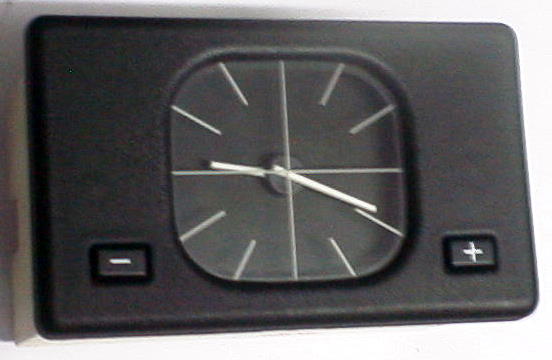The image depicts a matte black, rectangular desk clock with rounded edges, presenting a minimalist design. The clock's face is a square with similarly rounded edges, and it features no numbers, only lines indicating where the numbers would be, with a prominent plus sign stretching from top to bottom and left to right for the 12, 6, 3, and 9 positions. The clock is equipped with two white hands for the hour and minute indicators, with no second hand. Flanking the clock face, there are two buttons: a minus button on the left and a plus button on the right, both black with white symbols. The background of the image is stark white, and a shadow is visible in the upper left corner. There is also an indistinct light gray object partially cut out of the frame on the left side, potentially serving as a stand or background element.